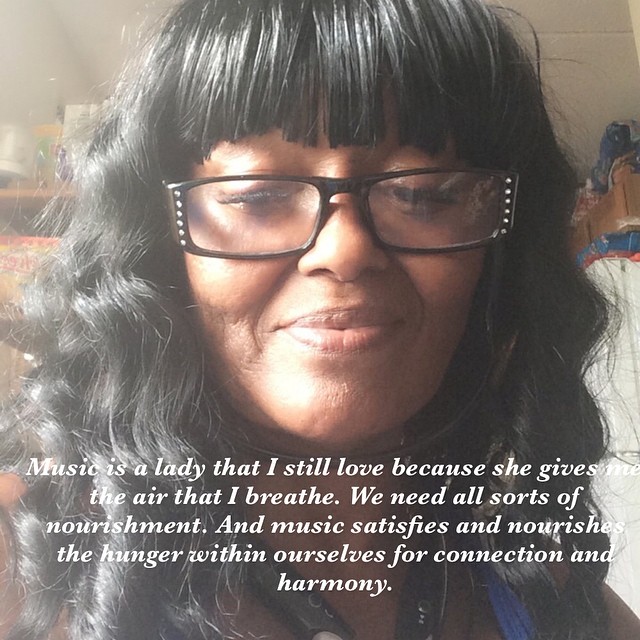The image features a woman with long, curly black hair that falls below her shoulders and bangs that cover her forehead. She is wearing black rectangular glasses and has headphones resting around her neck. The woman has dark skin and a sweet smile on her face as she looks down. Below her chin, in white italic text, it reads: "Music is a lady that I still love because she gives me the air that I breathe. We need all sorts of nourishment, and music satisfies and nourishes the hunger within ourselves for connection and harmony." She is dressed in a v-neck blouse with blue and brown colors. The background is indistinct, with unidentifiable objects partly visible and a wall behind her. The photograph is a square format, combining representational photography with graphic design and typography, filling about two-thirds of the image's height with the woman's face.